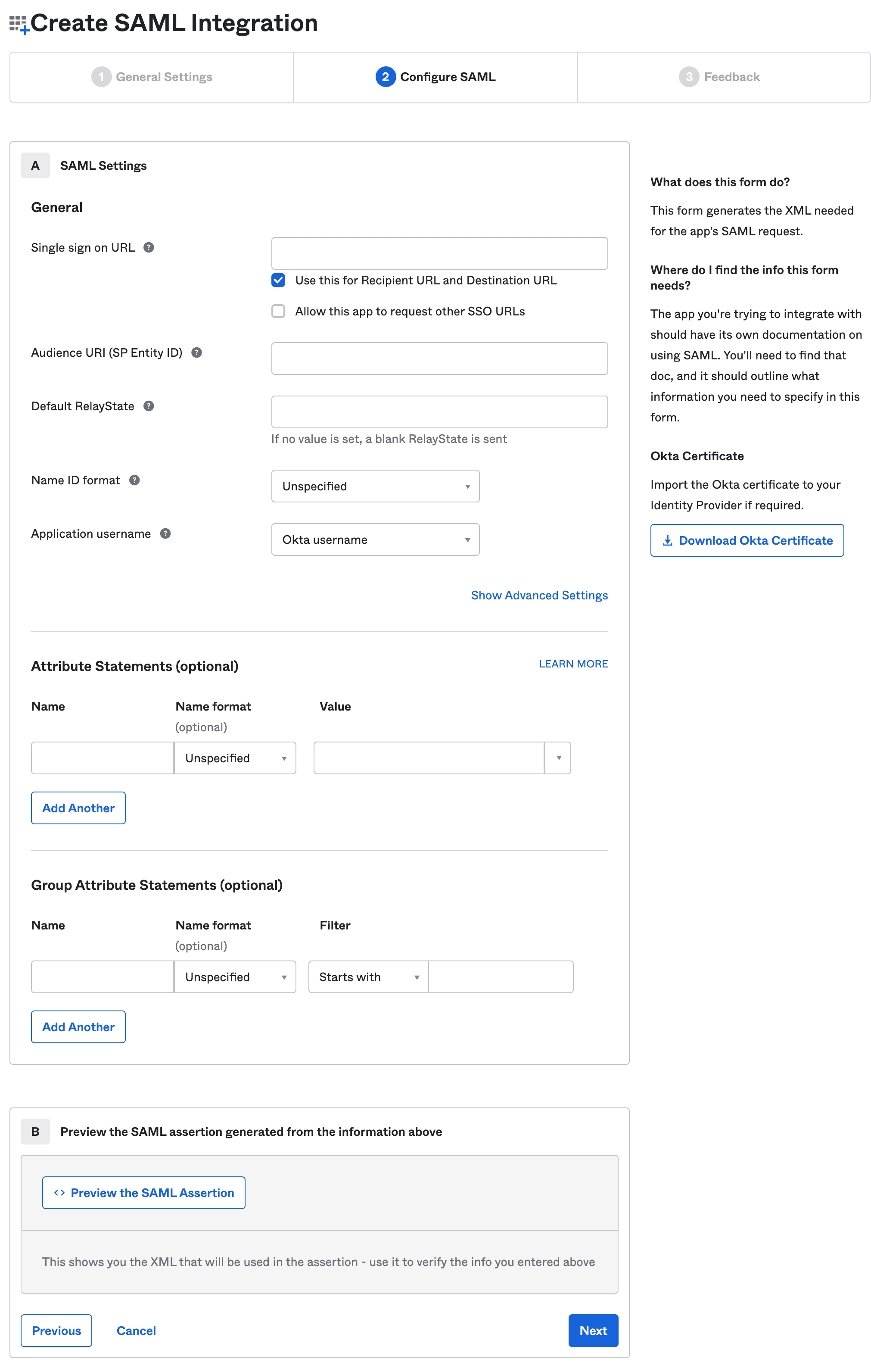Screenshot of the "Create SAML Integration" screen, part of a process for setting up Security Assertion Markup Language (SAML) authentication. SAML is a standard for identifying and authenticating users while enabling the transfer of these credentials to various service providers. 

In the image, a navigational interface with six squares is shown in the upper right corner. The bottom-right square features a plus sign and the text "Create SAML Integration." Below this, a sequence of steps is depicted, starting with "1. General Settings" in grey and "2. Configure SAML" highlighted, indicating the current step. Another step, "3. Feedback," is also displayed but is not highlighted.

The main section of the screen labeled "Configure SAML" includes text explaining the form's purpose, which is to generate the XML needed for the SAML request. Users are advised to consult the documentation specific to the app being integrated for the necessary information. There's also an option to "Download OKTA Certificate" for integration with the identity provider, marked by a blue rectangle with a download icon.

Below, "SAML Settings" are divided into sections:
- **Section A: Configuration**: Options include fields for "Single Sign-On URL," "Audience URI," "SP Entity ID," "Default Relay State," "Name ID Format," and "Application Username." There's a checkbox for using the recipient URL and destination URL, which is checked, and an unchecked box permitting the app to request other SSO URLs.
- **Attributes**: Customizable fields for "Attribute Statements" and "Group Attribute Statements" are available.

  Further down, **Section B** allows users to preview the SAML assertion generated from the configured information, verifying its accuracy.

At the bottom, "Previous," "Cancel," and "Next" buttons are available, with the "Next" button highlighted, guiding users to proceed to the following step.